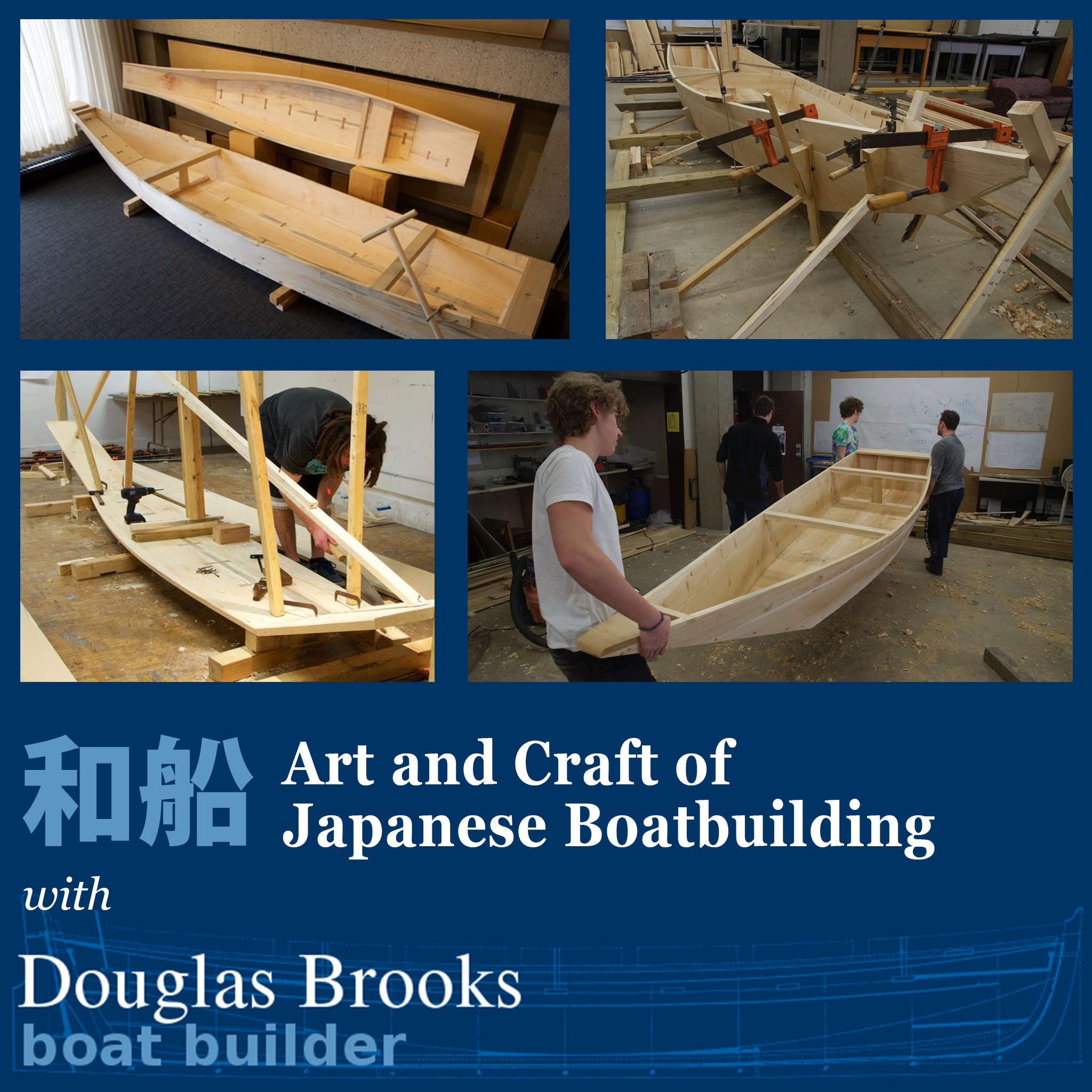The image represents the cover of a book or the title card of a documentary, featuring "The Art and Craft of Japanese Boat Building with Douglas Brooks, Boat Builder." Set against a dark blue background with Japanese text, it displays four photos that sequentially illustrate various stages of traditional Japanese boat construction. In the top left, a bare wooden outline of a boat begins to take shape. The top right shows the boat clamped and supported with wooden props, showcasing intricate craftsmanship. The bottom left captures the measurement phase on the workshop floor, scattered with wood shavings. Finally, the bottom right depicts three individuals carrying an almost complete boat, inspecting a blueprint on the wall. The boat, though structurally complete, awaits its finishing touches.